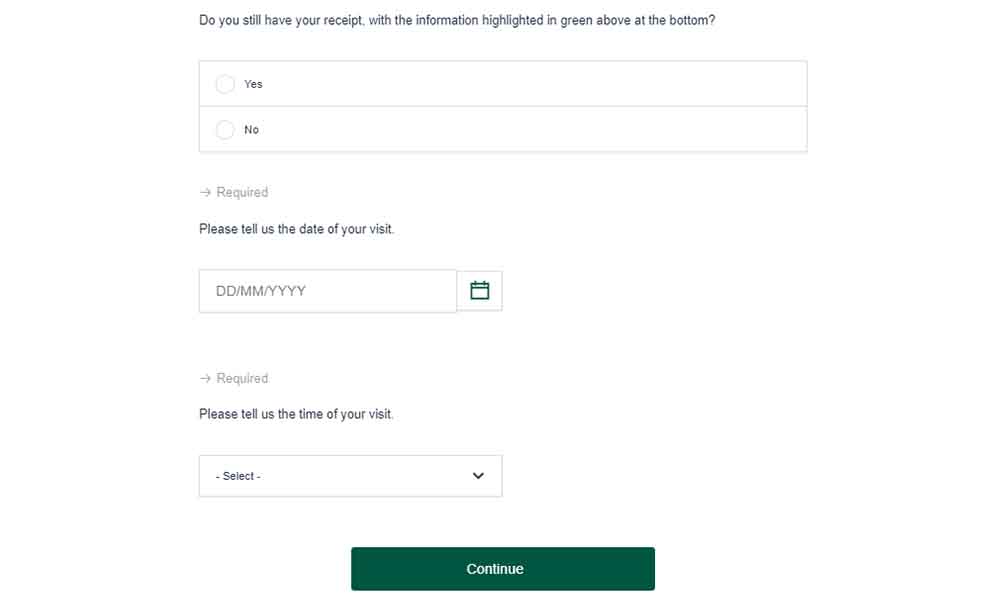This image is a cropped screenshot of a complaint section from a business website. The top part of the image is cut off, but the visible portion displays a form-like interface. At the bottom of the cropped section, there is a text prompt that reads, "Do you still have your receipt?" with the words "information highlighted in green above" absent due to the crop. Below this prompt, there is a large rectangular box offering two circular options for selection: "Yes" on top and "No" below. Neither option is currently selected.

Further down, in small gray print, the word "Required" appears. Following this, a bold black prompt reads, "Please tell us the date of your visit," accompanied by a large date input box. Inside the date box, there is placeholder text "DDMMYYYY" and a calendar icon situated to the right. Again, the word "Required" appears in small gray letters underneath.

Next, another bold black prompt asks, "Please tell us the time of your visit," accompanied by a dropdown box. Inside the dropdown box on the left side is the word "Select." 

Centered at the bottom of the screenshot is a large green bar featuring the word "Continue" in small, white font.